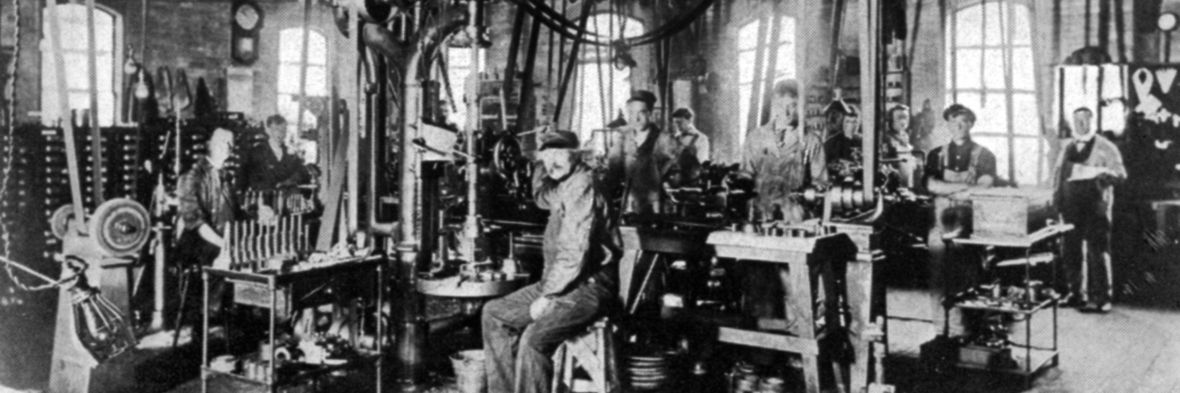In this black and white photograph, a bustling early 20th-century factory setting is captured in striking detail. The factory floor is populated predominantly by men, with a few women also present, all clad in period-appropriate work attire. They are either seated or standing at various desks, intently focused on the camera. The factory is brimming with antiquated machinery, whose exact function remains ambiguous, though it suggests a production line of either mechanical or fabric nature. Overhead, cords and pipes dangle from the ceiling, adding to the industrial ambiance. The workspace is well-lit by several large windows, and a clock on the wall hints at the meticulous timing essential for such manufacturing operations. The array of machinery, combined with the workers' attire and the photo's grayscale tone, evocatively harks back to the nascent era of industrial manufacturing.